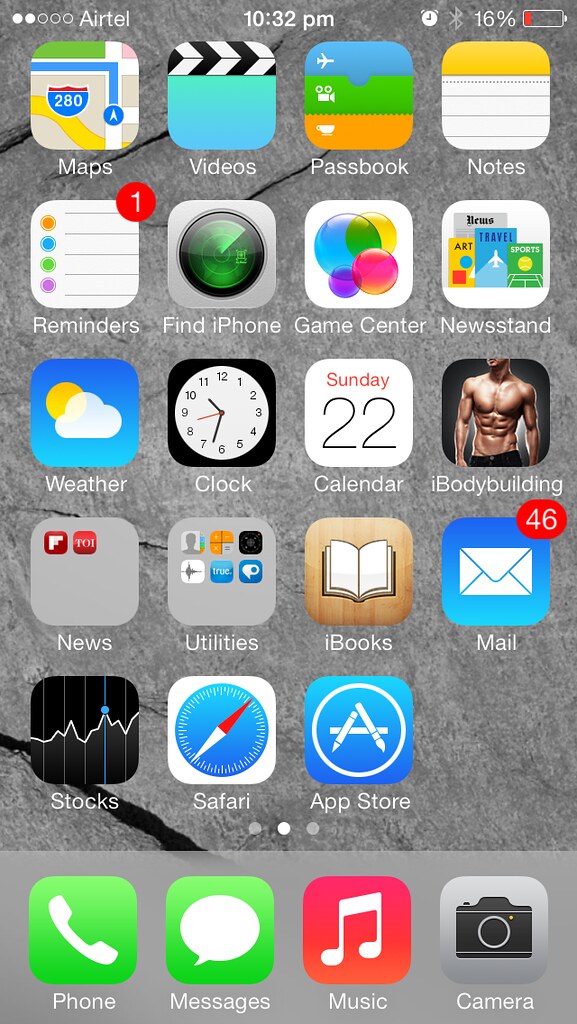This is a screenshot capturing the home screen of an iPhone. At the top, the status bar displays 2 bars of signal strength for the Airtel network, with the current time indicated as 10:32 p.m. Alongside, there are icons for alarm, Bluetooth, and a battery icon showing 16% charge remaining.

The screen is populated with several apps arranged in rows. The first row contains the Maps, Videos, Passbook, and Notes apps, each distinguished by their respective colors. The next row features the Reminders app, with a red badge indicating one pending reminder, followed by the Find iPhone, Game Center, and Newsstand apps.

Beneath them, the Weather, Clock, and Calendar apps are visible, along with an app related to bodybuilding. There are also folders named News and Utilities, alongside the iBooks app. Moving further down, the Mail app displays 46 unread emails, and the dock section at the bottom of the screen includes the Phone, Messages, Music, and Camera apps.

The detailed arrangement reflects a typical user's organization of their essential applications and tools on their iPhone's home screen.